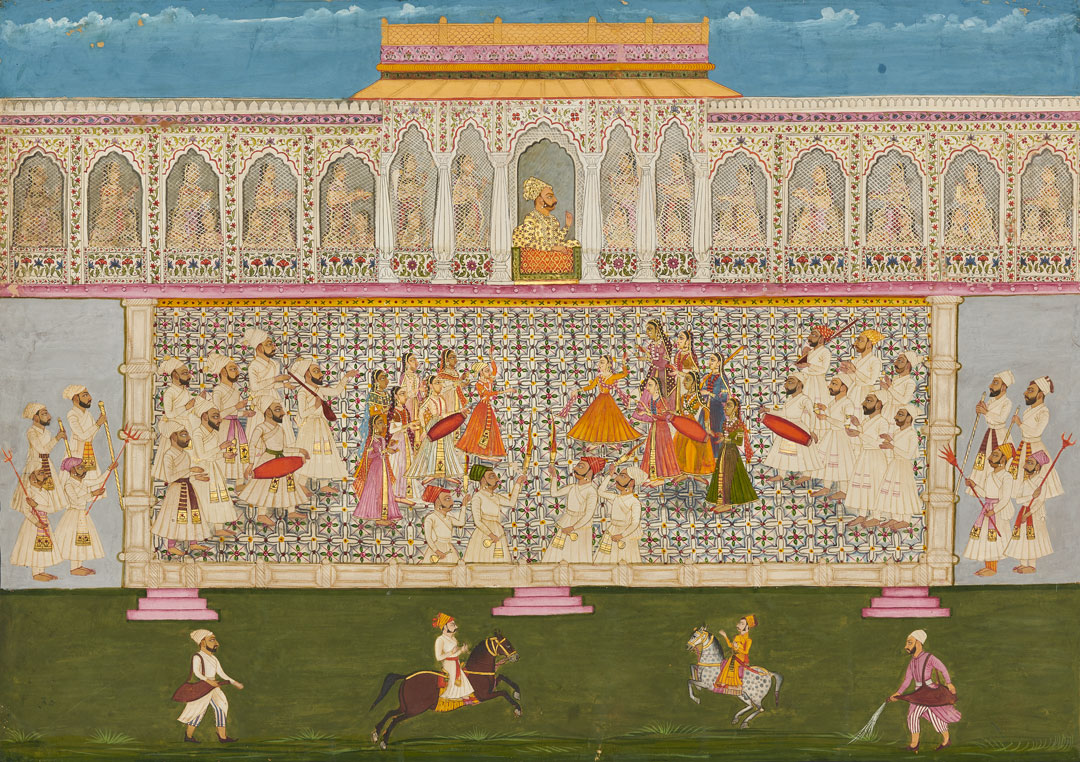This painting, evocative of traditional Indian or Hindu art, depicts a bustling and intricate scene with a somewhat flat perspective. Dominating the background is a grand, rectangular palace with a blue sky above. At the top of the building, there's a series of windows or arches, and within each, women dressed in vibrant colored gowns—yellow, blue, green, and pink—are visible, often adorned with headdresses and possibly peering through mesh screens.

Central to the composition is a man standing on a balcony, characterized by his distinctive handlebar beard and surrounded by the building's sumptuous golden rooftop. Below this upper section, set within the palace walls, the scene is densely populated with men mostly in white robes and headscarves, some carrying swords or instruments, flanking a group of women. This ensemble appears to be engaging in a social or courtship ritual within a courtyard setting.

At the bottom of the painting, a grassy expanse hosts additional figures involved in various activities. Two individuals are mounted on horses, while others are watering the grass using sheepskin containers. The scene is rich with cultural detail, capturing a moment of dynamic interaction and vibrant attire against the backdrop of an elaborately adorned palace.